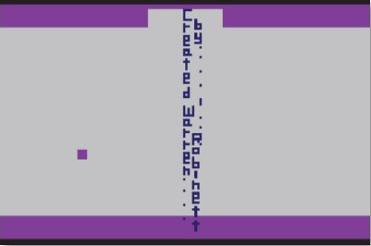This image resembles a rudimentary computer game from the early 1980s. It features a grey background with two horizontal purple strips—one at the bottom and one at the top. The top strip is interrupted by vertical text that reads "created by," with "created" spelled out in blue lowercase letters aligned top-to-bottom. To the right of this, the word "by" is very faintly visible, followed by "robinette" beneath it. Additionally, on the grey background to the left of the bottom purple strip, there is a solitary purple square. The entire design maintains a simple, vintage aesthetic typical of early digital graphics.